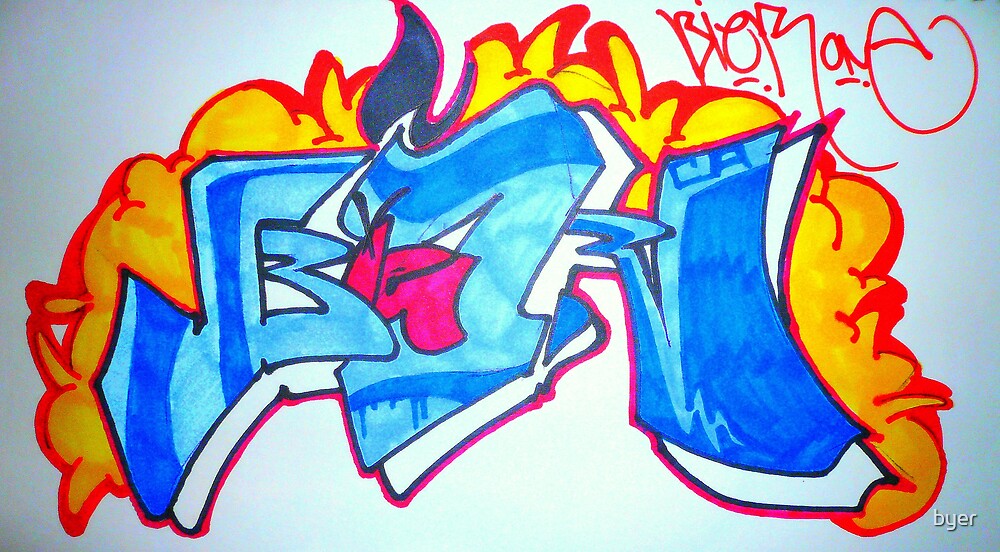This vibrant, graffiti-style illustration features a dynamic composition of multi-colored elements and cryptic text, suggesting it may have been created on a canvas or paper. Dominating the image is a horizontal array of blue letters, intermixed with a smaller magenta letter, all outlined in black with a 3D effect in white to the right. The letters sit atop a cloud-like orange mass, accented in red, and surrounded by flames. The vivid colors include shades of red, pink, yellow, light and dark blue, gold, and orange, set against a grayish background that darkens toward the edges. In the top right corner, an artist’s signature in red—possibly reading "B-I-O" or "K-O-E"—adds a personal touch to the piece, while a watermark in small white text at the lower right corner states "Bayer."